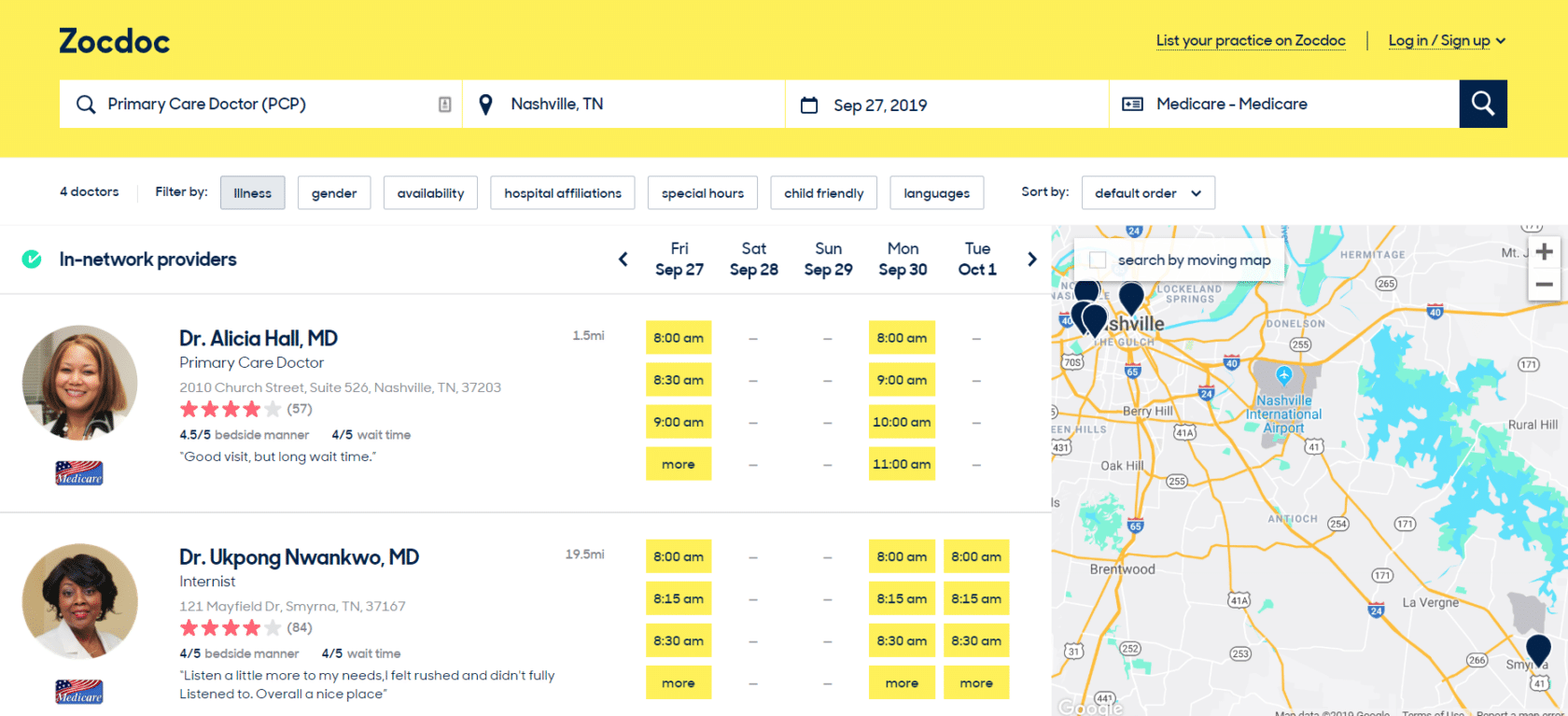This is a detailed screenshot from the ZocDoc website. At the top of the page is a prominent yellow banner. The ZocDoc logo is displayed in black letters on the top left, while the top right features options to "List your practice on ZocDoc" and "Log in/Sign up." Below this is a selectable menu for finding healthcare providers, with fields pre-filled for "Primary care doctor" and "PCP" in "Nashville, Tennessee," along with the date "September 27, 2019" and the insurance type "Medicare-Medicare."

The page offers filtering options by illness, gender, availability, hospital affiliations, special hours, child-friendliness, languages, sorting by default order, and in-network providers. 

The first listed provider is Dr. Alicia Hall, MD, a primary care doctor located at 2010 Church Street, Suite 526, Nashville, Tennessee, 37203. She has 4 out of 5 stars based on 57 ratings, a bedside manner rating of 4.5 out of 5, and a wait time rating of 4 out of 5, though one patient noted "good visit but long wait time." Her office is 1.5 miles away, with available slots on Friday, September 27 (8:00 AM, 8:30 AM, 9:00 AM), none on September 28-29, but appointments available on Monday, September 30 (8:00 AM, 9:00 AM, 10:00 AM, 11:00 AM).

The second provider listed is Dr. Akpong Nwankwo, MD, an internist situated at 121 Mayfield Drive, Smyrna, Tennessee, 37167. He also holds a 4 out of 5 star rating from 84 reviews, with ratings of 4 out of 5 for both bedside manner and wait time. One review stated, "listen a little more to my needs, I felt rushed and didn't fully listen to, overall a nice place." His practice is 19.5 miles away, offering availability on Friday, September 27 (8:00 AM, 8:15 AM, 8:30 AM), and no slots on September 28-29, but available on Monday, September 30 (8:00 AM, 8:15 AM, 8:30 AM), and Tuesday, October 1 (8:00 AM, 8:15 AM, 8:30 AM).

To the right of this information, there is a map pinpointing multiple locations in Nashville where these practices are situated.